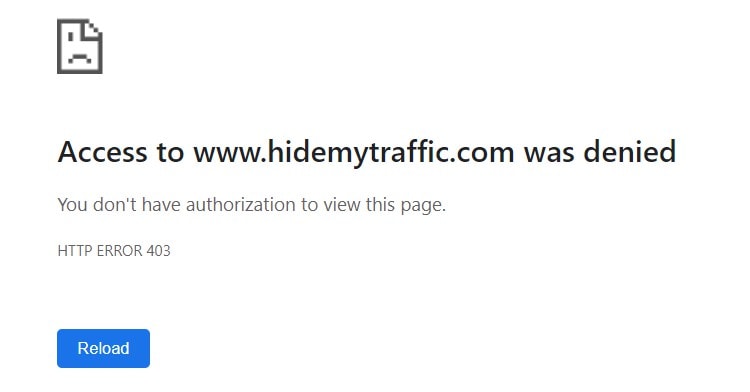The image depicts a minimalistic webpage displayed on a white background with no borders. In the upper left-hand corner, there is a square icon outlined in gray, featuring a frowny face with one corner folded over, suggesting a page error. Directly beneath this icon, bold black text states, "Access to www.hidemytraffic.com was denied." Further down, smaller, gray text clarifies with, "You don't have authorization to view this page." Below this message, capitalized black text reads, "HTTP ERROR 403." Finally, at the bottom, there is a bright blue button with "RELOAD" written in white text. The overall design is simplistic and straightforward, emphasizing the access denial and error status.